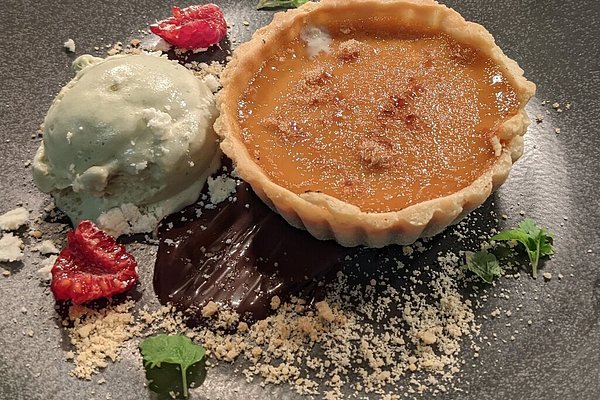In this detailed image, we see a beautifully presented dessert, likely from an upscale restaurant, arranged on a dark, speckled plate that could be black, brown, or dark gray. Dominating the plate is a caramel-colored tart or possibly a creme brulee, its enticing crust promising a delightful crack when pierced. Adjacent to the tart, on the left side, sits a generous scoop of off-white ice cream—perhaps vanilla, butter, or even light green pistachio. Flanking the ice cream are two halved raspberries, adding a vibrant pop of red. Beneath the tart and ice cream is a smear of rich, hardened chocolate or chocolate fondue. The plate is artistically garnished with a few fresh sprigs of parsley or mint, and scattered cookie crumbs or dessert crumbles that add texture and visual appeal. There is no text overlay on the image, allowing the viewer to fully appreciate the meticulous and appetizing presentation.